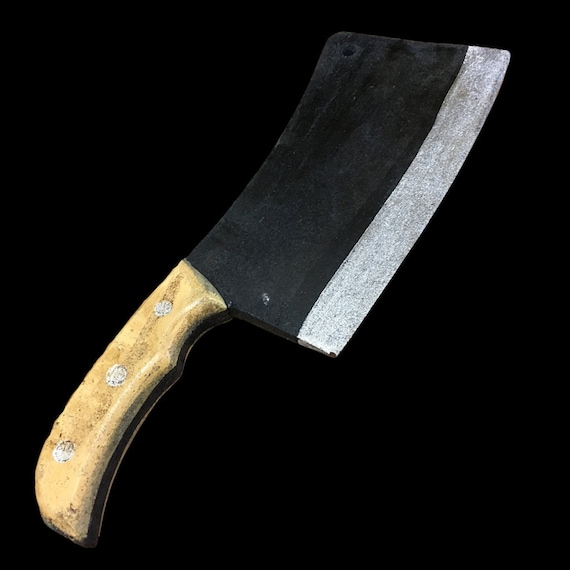This square-shaped image prominently features a large meat cleaver against a solid black background. The cleaver boasts a substantial, almost matte black blade with a sharp cutting edge that gleams silver. Near the edge, the blade transitions to a light gray color. The cleaver's top part, near the handle, includes a distinctive round hole. 

The handle of the cleaver is light brown wood, secured with three grayish screws, indicating signs of use. The black stripe running down through the handle adds to its rugged appearance. The cleaver is positioned with its handle pointing towards the bottom left corner and the blade's sharp edge directed to the right, emphasizing its formidable size and sharpness.